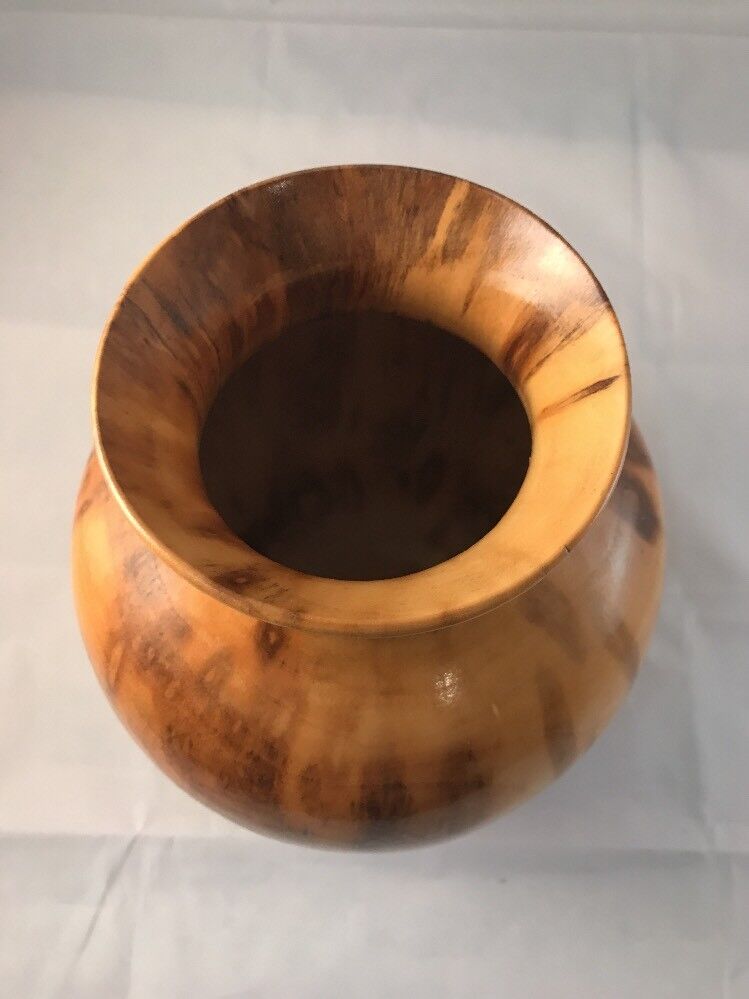The image is a vertical rectangular photograph of a tall, wooden pot or urn, viewed from the top down at a slight angle, showcasing its wide mouth and bulbous, tapering form that flares out again towards the base. The wood is smooth and exhibits a rich grain, featuring various shades of brown with golden hues and darker streaks, including a prominent dark streak on the right side. This pot sits on a white, wrinkled surface, likely a tablecloth. The dark interior of the pot is empty, adding a sense of mystery to its function, which could range from transporting food or seeds to serving as an artifact. The intricate wood grain and the pot's unique shape contribute to its beautiful, striking appearance.